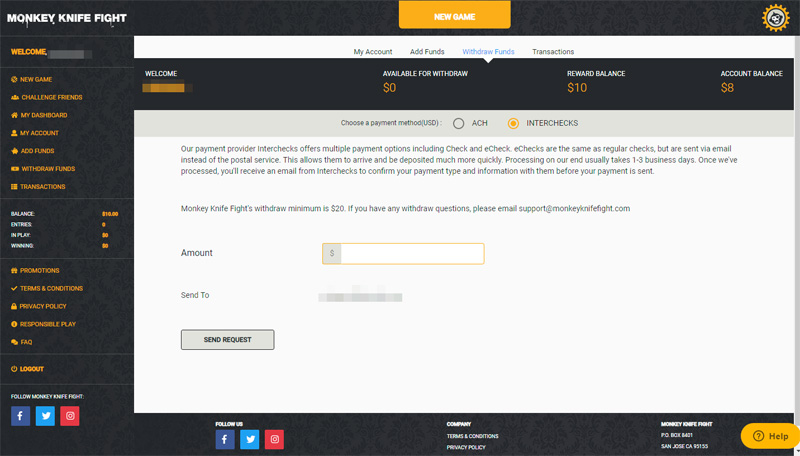The website for Monkey Knife Fight features a navigation bar with several important options and information at the top. At the top left, there's a prominent "New Game" button, inviting users to try the latest gaming options. In the top right corner, there's an intriguing symbol adorned with yellow rays, possibly representing sunlight or energy.

Upon logging in, the user is greeted with: "Welcome," though this message briefly flashes before their eyes. The account management section includes options like "Add Funds," "Withdraw Funds," and "Transactions." The account summary indicates an available withdrawal balance of $0, a reward balance of $10, and an overall account balance of $8.

Payment options are prominently displayed, detailing methods like ACH and Interchecks. Interchecks provides multiple payment avenues such as link checks and e-checks, which function similarly to regular checks but can be processed and deposited more swiftly. Typically, processing and arrival of payments take about 1-3 business days. Users will receive an email from Interchecks to confirm payment details within a 45% processing window. 

The website notes that the minimum request for a trial is $20. For any support or questions, users are directed to email support@monkeyknifefight.com.

Additional menu items on the site include "Challenge Runs," "My Dashboard," "My Account," "Entries in Play," "Winnings," "Promotions," "Terms and Conditions," "Privacy Policy," "Responsible Play," "FAQ," and "Logout."

At the bottom of the site, users are encouraged to follow Monkey Knife Fight on social media, indicated by blue and red square icons, possibly linked to different social platforms. The company details, including "Terms and Conditions" and "Privacy Policy," are also outlined, and it appears the company is based in San Jose, California.